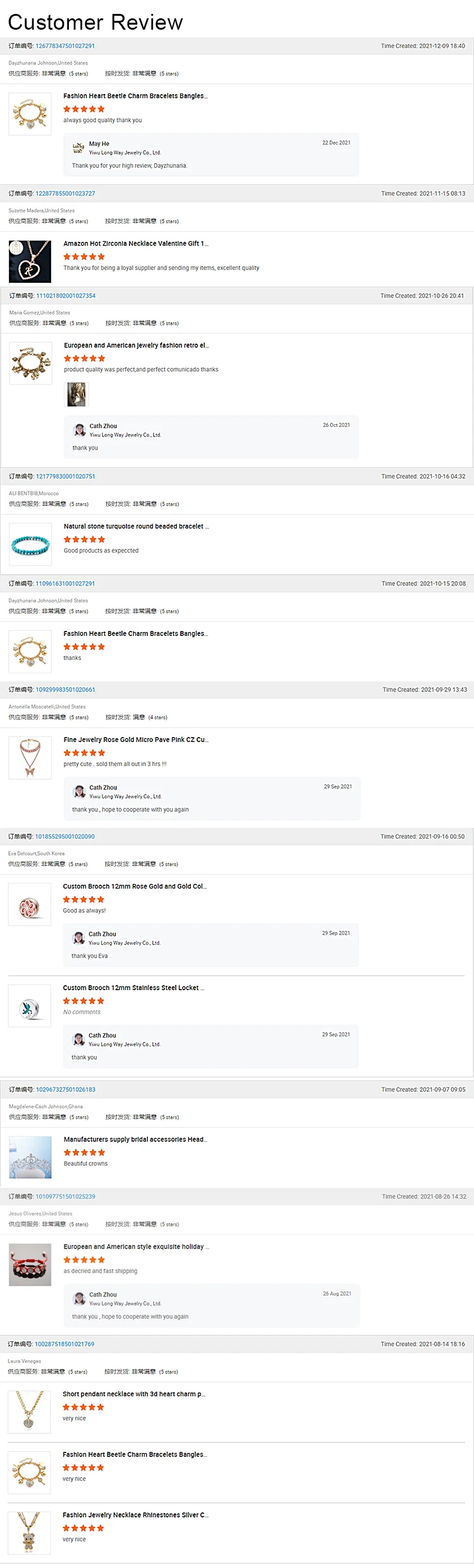Screenshot of Customer Reviews on Mayhee's Website

This screenshot captures the customer review section of Mayhee's website, showcasing a series of positive feedback on various jewelry items. The most recent review, posted on December 9, 2021, at 6:40 PM, features high praise for the "Fashion Heartbeetle Charm and Bracelet Spangle." In response, Mayhee has expressed their gratitude with a message: "Thank you for your high review."

Descending the page, the reviews become older, with the next one dated November 15, 2021, at 8:13 PM. All reviews on this page are rated five stars and share a common sentiment, stating "very nice." Mayhee has responded to each one with a simple "thank you," showing consistent engagement with their customers.

The jewelry pieces being reviewed appear highly realistic, predominantly showcasing a lustrous gold color. The company's dedication to quality and customer satisfaction is reflected in the uniformly positive feedback and their thoughtful acknowledgments.